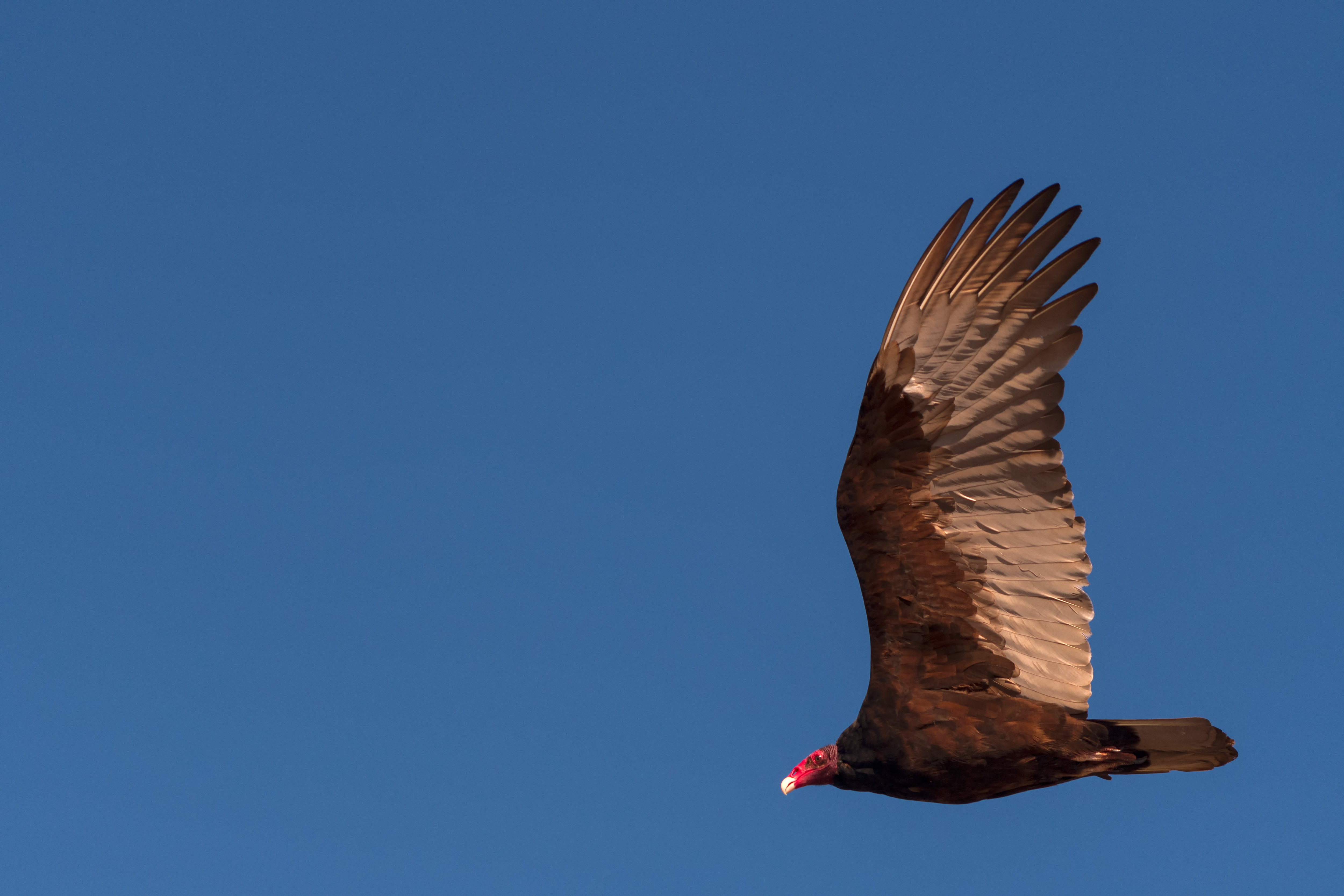A large bird, likely a buzzard or vulture, soars horizontally from right to left against a pristine, cloudless blue sky, positioned in the lower right-hand corner of the image. It is captured in the upstroke of its flight, showcasing one outstretched wing that stands almost vertical to its body. The bird's red-colored head and white beak contrast strikingly with its dark brown feathers, which cover its body and the upper sections of its wings, transitioning to a lighter brown on the lower portions. Its legs and talons are hidden, tucked closely against its body. The sky's flawless blue hue seems almost surreal, enhancing the bird's impressive figure mid-flight.